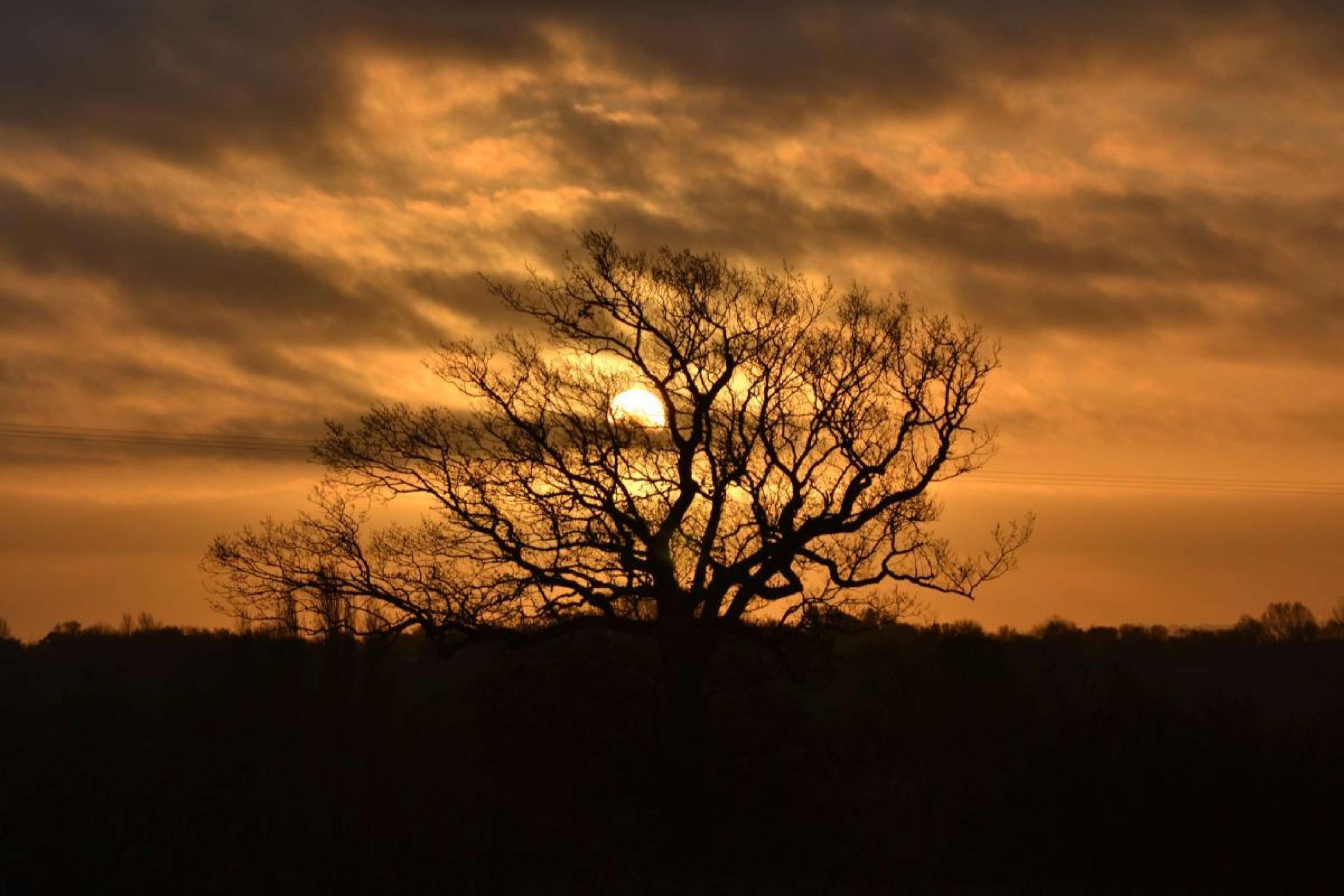The photograph captures a moody, Old West-inspired scene at sunset, emphasizing a spindly, barren tree or large bush that dominates the foreground. The tree, devoid of leaves, stretches its wide, intricate branches against a backdrop of a darkening sky, rich with golden and hazel tones. The sunset casts an orange glow, partially obscured by dark gray clouds that reflect the waning daylight. Shadows of the grass underneath the tree blend seamlessly into the photo's lower half, forming a stark, black silhouette against the luminous, deserty horizon. The overall atmosphere is simple yet evocative, bathed in the muted, golden hues typical of a desert twilight, evoking a sense of timeless solitude.